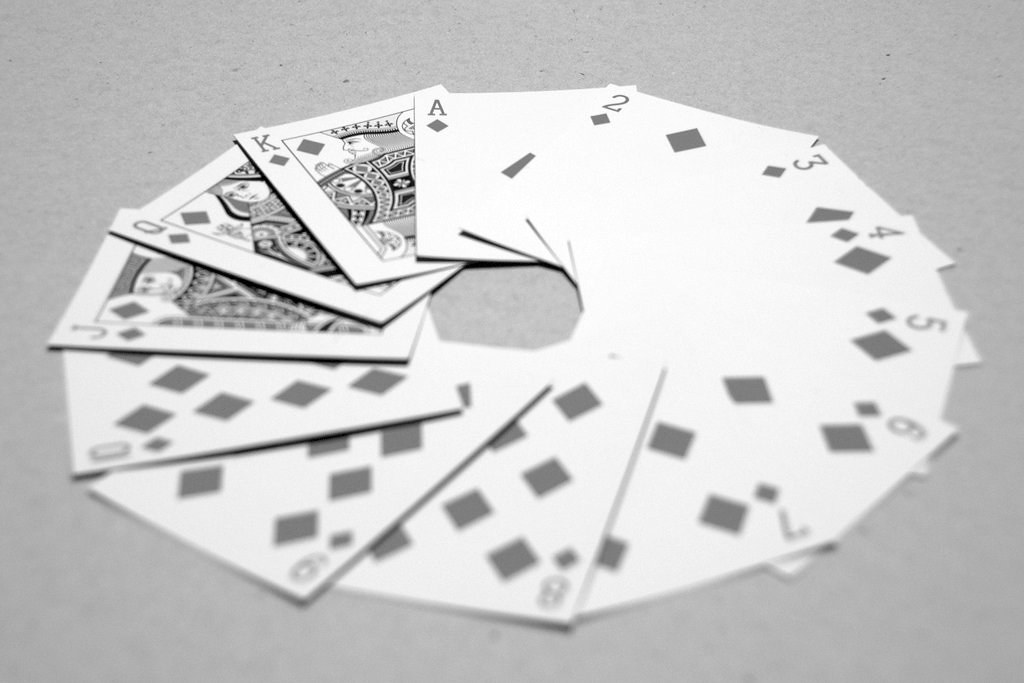In this black and white image, the textured, grainy gray background evokes a sense of a rocky, pebbly surface. The varying light sources and shadows create a mesmerizing gradient of gray tones, with darker shades accentuating the corners and lighter hues illuminating the central area. The bottom left and right corners exhibit a subtle blur, contrasting against the sharper upper portion.

At the center of the image lies an intriguing arrangement of 13 playing cards, meticulously spread out in a circular formation. Starting with the two of diamonds, each subsequent card follows sequentially through to the ace of diamonds, all layered gracefully on top of one another. This thoughtful arrangement creates an empty space in the middle of the circle, enhancing the visual appeal and inviting closer examination.